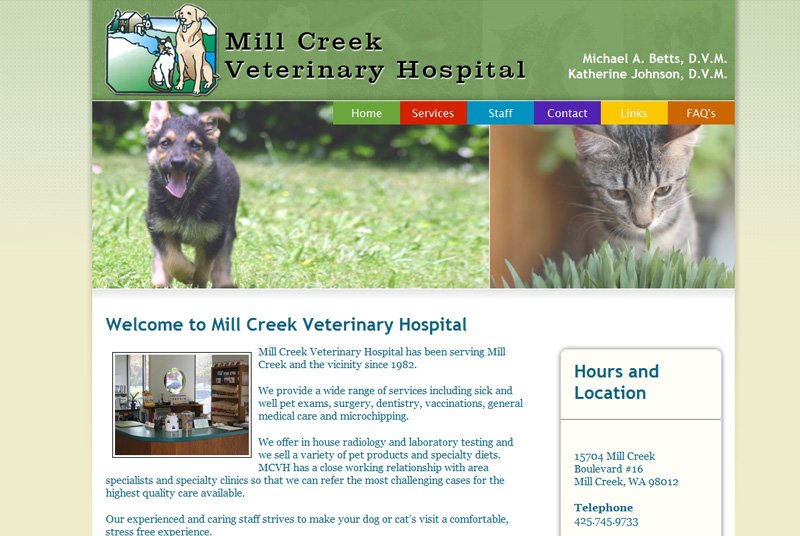Welcome to the Mill Creek Veterinary Hospital website, a comprehensive online portal showcasing the full spectrum of services offered at this dedicated pet care facility. Located at 15704 Mill Creek Boulevard, Number 16, Mill Creek, Wisconsin, 98012, the website provides detailed information about their offerings, including pet exams, surgeries, dental care, vaccinations, medical care, and microchipping. The hospital is equipped with advanced radiology and laboratory testing services, and also offers a selection of pet products and specialty diets.

The homepage features a welcoming banner with images of a dog running joyfully in the sun and a curious cat peering down at a plant, creating a friendly atmosphere for pet owners. Visitors can easily navigate to different sections of the site, marked in various colors: Home, Services, Staff, Contact, Links, and FAQs. The website highlights the hospital's commitment to providing high-quality care for pets and underscores their collaborative relationships with area specialists for handling the most challenging health cases.

Additionally, users can find essential contact information, including phone numbers, and a schedule of operating hours. The prominently displayed visuals and intuitive layout make it easy for pet owners to feel connected and informed.